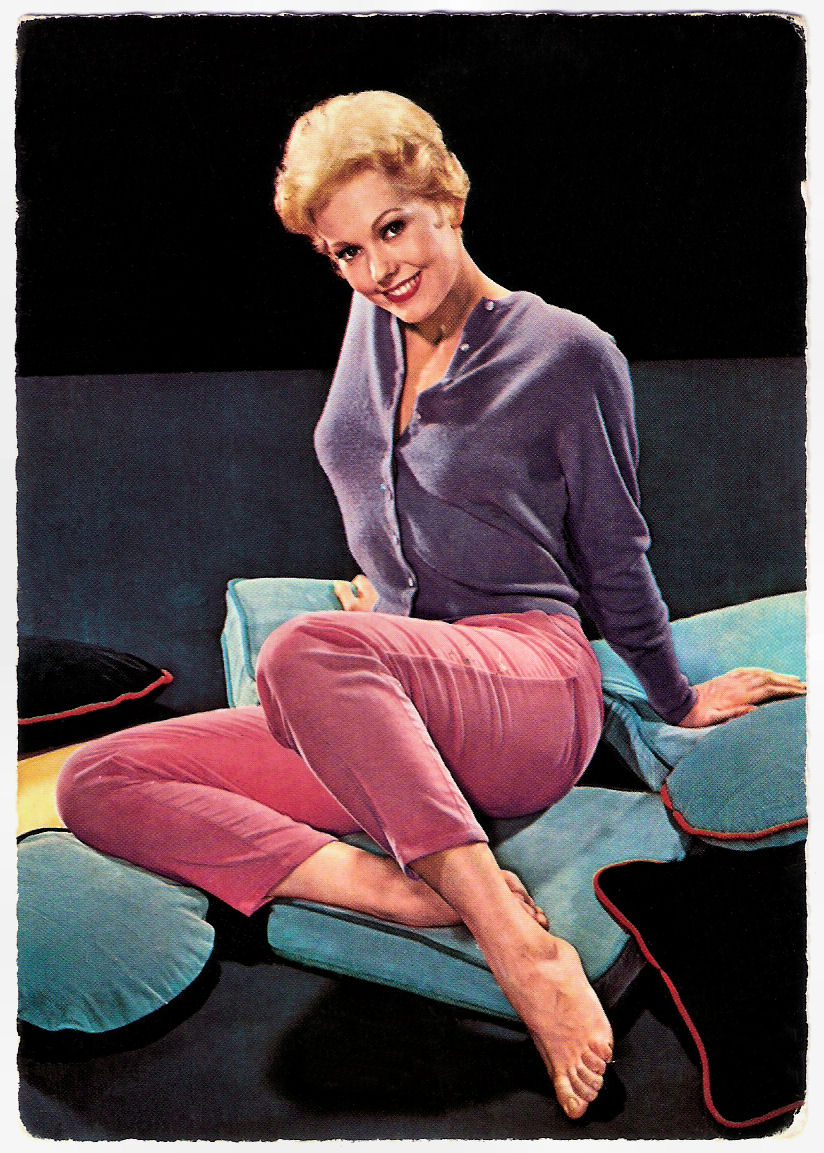In this photo of Kim Novak, she sits on a series of cushions on what appears to be a dark, likely gray or dark blue, floor or carpet. She's dressed in pink jeans that reach mid-calf and is barefoot. Her upper clothing consists of a purple button-up blouse, casually unbuttoned halfway down her chest, revealing some skin. Kim supports herself with both hands resting on a mix of aqua green and black cushions. Her short blonde hair complements her red lipstick, giving her a classic look. She poses with her body slightly leaning to the left and her legs bent, with one leg more pointed toward us while the other bends to her side. Behind her, the background is entirely pitch-black, amplifying the focus on her. The image has a worn-out, cutout aesthetic, reminiscent of a torn magazine photo, particularly noticeable along the top edges where signs of wear are visible. Her expression is inviting, with a tilted head and a smile aimed directly at the viewer.